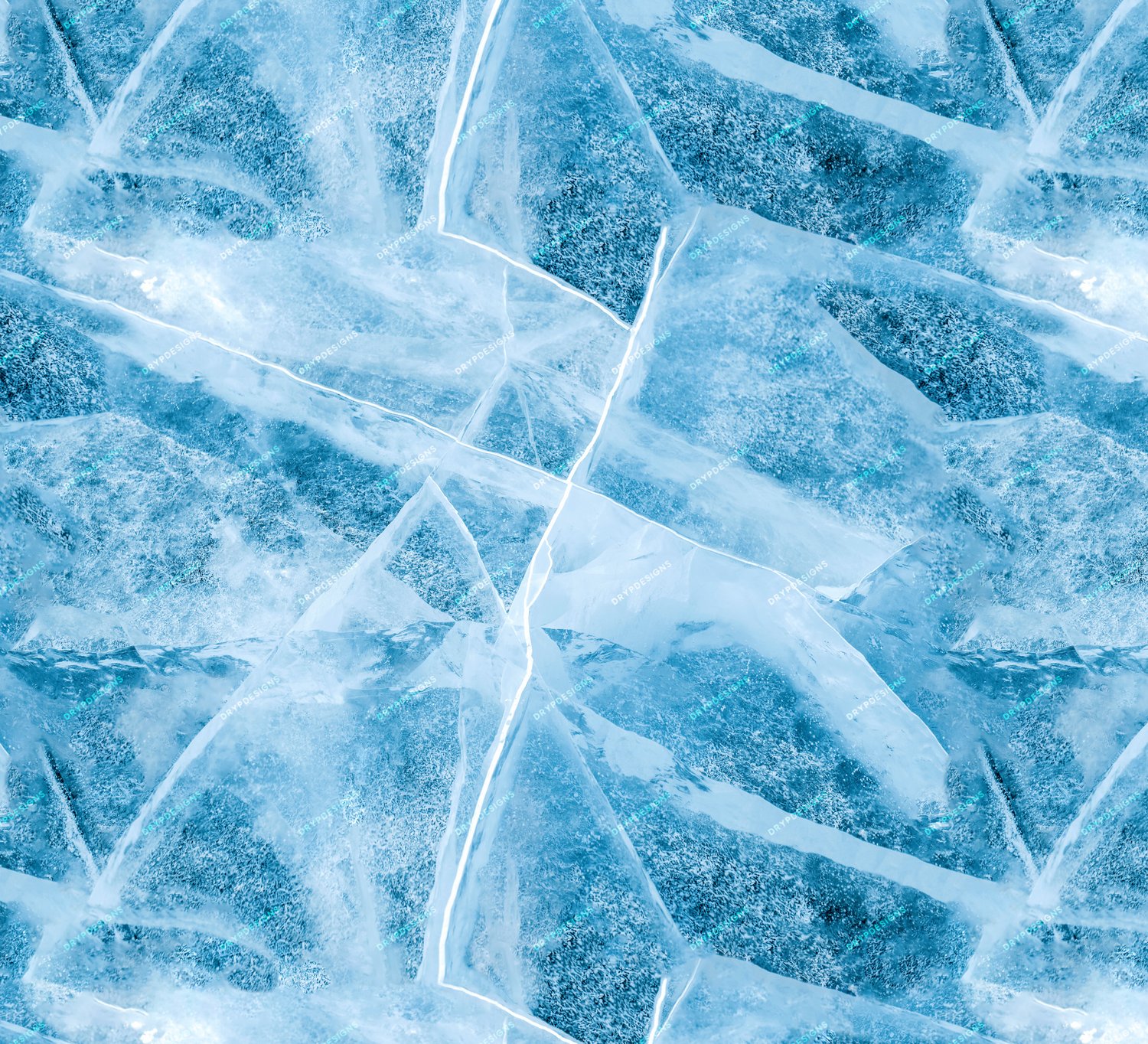This image features an intricate background of varying shades of blue, ranging from dark to light and intermixed with hues of white. Streaks of white lines traverse in all directions across this blue canvas, originating from the lower center and fanning out towards the left center, then looping back up to the top center. These white lines create a network of intersecting paths, with one notable intersection at the upper left portion of the image. The lines extend fluidly from the left center down to the bottom right, reminiscent of delicate, wispy clouds that diverge from the more pronounced white streaks.

Visually, the scene evokes the appearance of cracked or broken ice on a thick, frozen pond. It mirrors the splintering effect that occurs when ice begins to crack beneath one's feet without fully giving way, revealing the dark blue underside of the ice. The fractures are lighter in color, contributing to a textured, patterned effect. This motif of cracked ice is repeated vertically, with identical elements present at both the top and bottom of the image, enhancing the sense of symmetry and continuity throughout the scene.